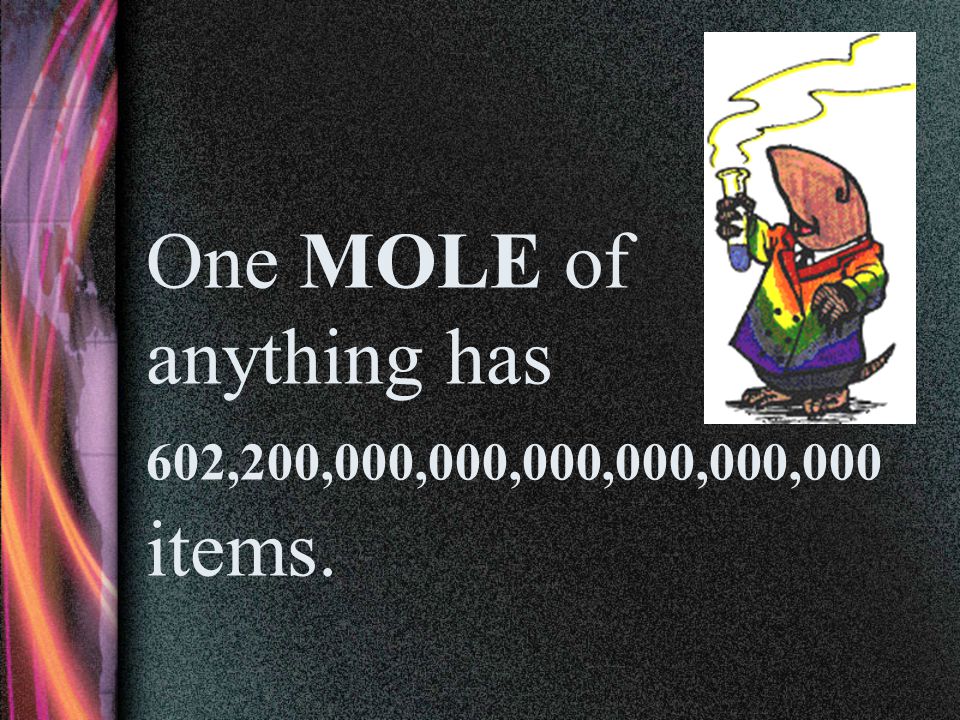This image appears to be a slide from an educational PowerPoint presentation. The background features a grainy black texture with a thin vertical strip on the left side, occupying about one-tenth of the slide. This strip displays a stylized, purple globe with black oceans, overlaid with various pink lines. Centered on the black background is a piece of white text that reads, "One mole of anything has 602,200,000,000,000,000,000,000 items." In the top right corner of the slide, there is a cartoonish, humanized mole. The mole is depicted standing on its hind legs, wearing a vibrant rainbow-colored lab coat, and holding a beaker with smoke or fumes emanating from it. The mole's attire and the overall colorful palette, which includes shades of pink, purple, red, orange, green, black, and white, enhances the engaging and whimsical educational tone of the slide.